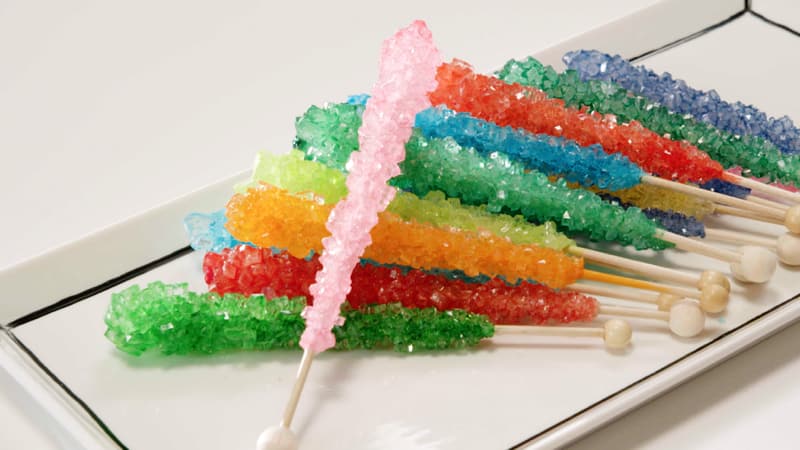This photograph showcases an array of Rock Candy sticks elegantly arranged on a white tray with black lines outlining its edge. The tray is centered in a backdrop of light gray, emphasizing the vibrant colors of the candy. Each Rock Candy stick features a long, crystallized section attached to a stick that varies from cream to light brown in color. At the bottom of every stick, there's a round ball in either white or beige, providing a sturdy base. The candy crystals themselves come in an assortment of colors, including light pink, lime green, forest green, orange, red, yellow, light blue, blue, and purple. In total, 10 to 15 candy sticks are meticulously organized in rows, with a notably upright pink one standing out. The crystallized sections stretch nearly the entire length of the sticks, giving them a full and ornate appearance.